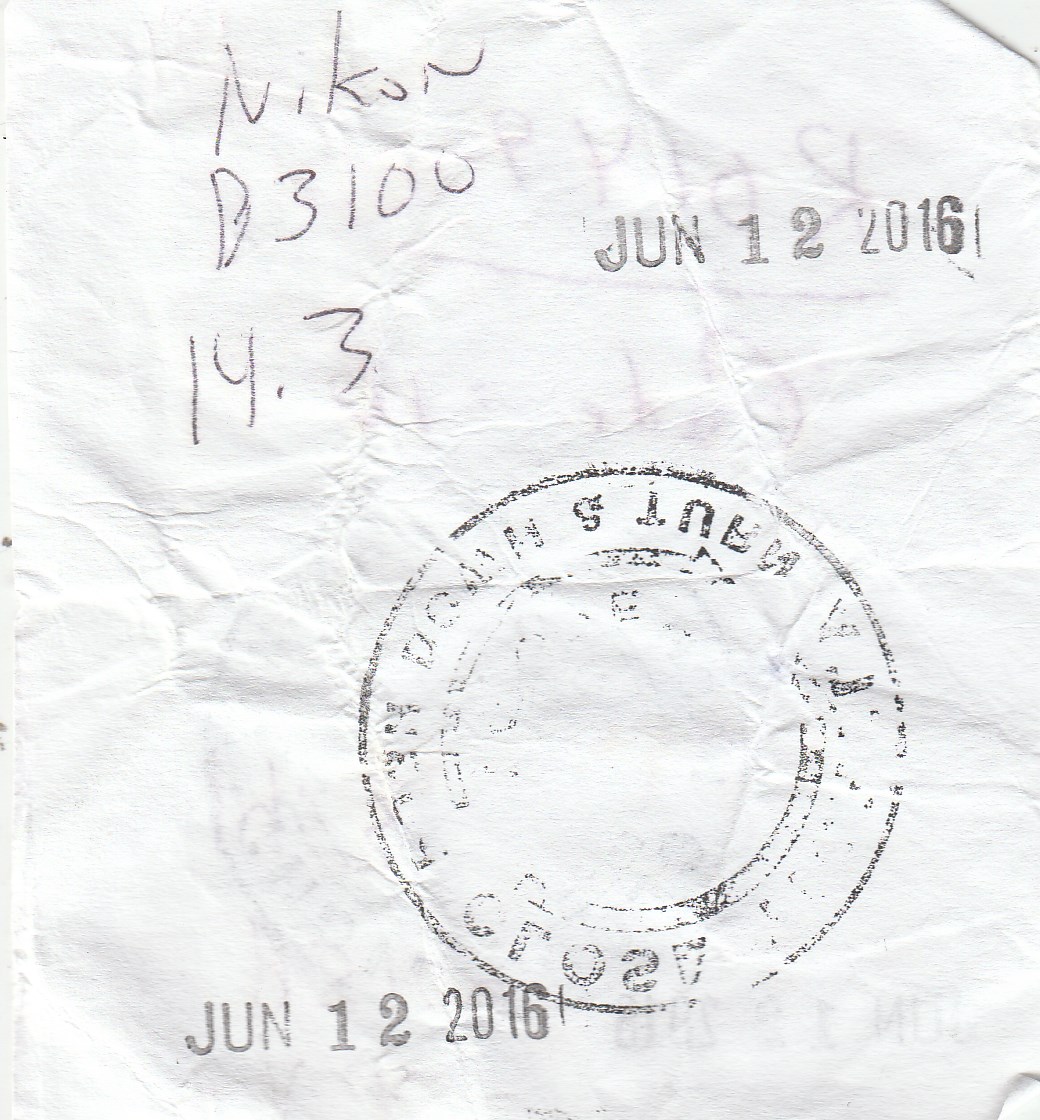The image portrays a slightly vertically oriented photograph of a receipt or a piece of paper characterized by a combination of stamps and handwritten elements. In the upper left-hand corner, the word "Nikon" is meticulously handwritten in black ink, following the brand's stylization. Directly underneath "Nikon," the model designation "D-3100" is written, followed by the figure "14.3." Adjacent to this text, a distinct date stamp reading "JUN 12, 2016" is positioned prominently, with an identical stamp mirrored in the bottom left corner of the paper. Centrally placed between these two date stamps is an indistinct circular stamp, reminiscent of a type used by passport control officers, adding an element of officialdom or verification. The paper exhibits signs of potential folding, suggesting that it might have been handled frequently, and there are hints of additional text bleeding through from the reverse side. Overall, the image captures a piece of paper ingrained with personal annotations and formal date markings, evoking the feel of casually noted information on a convenient scrap of paper.